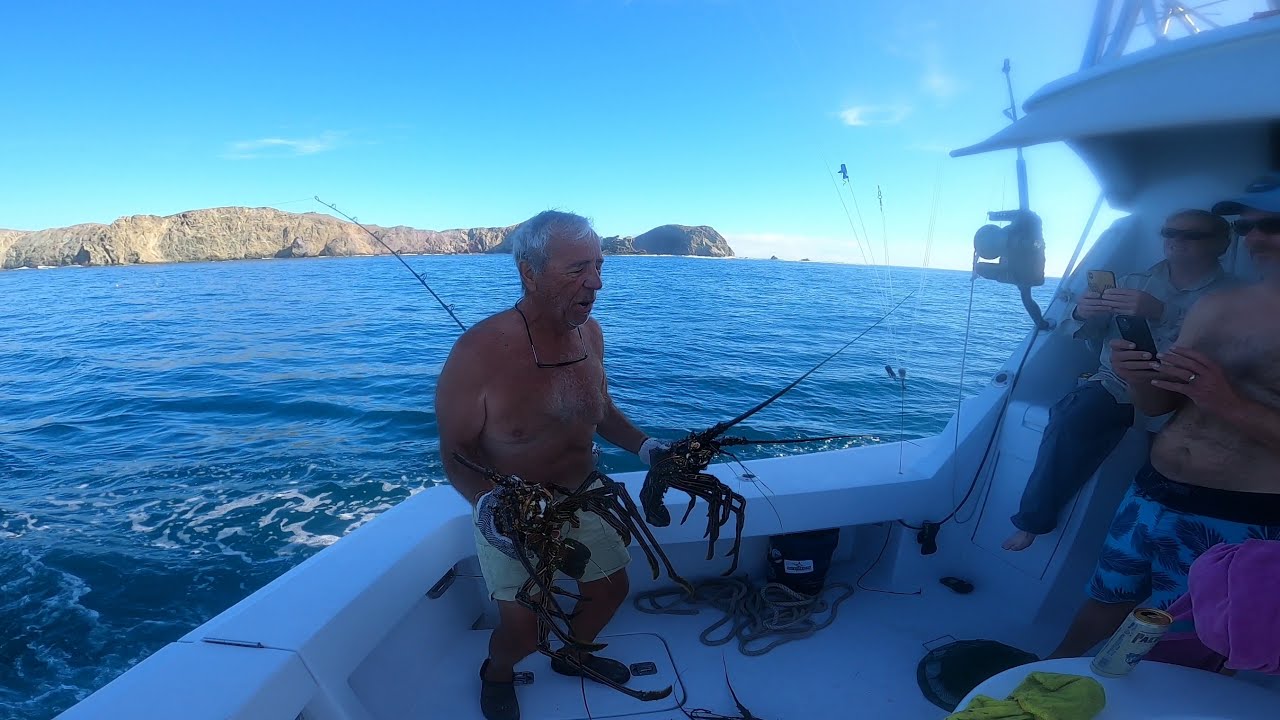In this vivid outdoor scene, a fresh catch moment is captured on a white fishing boat. Anchored against a backdrop of clear blue sky and gleaming rocky cliffs, an older, shirtless man stands prominently in the center of the image. His gray hair hints at his age, and he wears a pair of yellow swim trunks as he proudly showcases two lobsters, held with gloved hands for safety. Behind him, the fishing pole is mounted on the boat. On the boat’s right side, two individuals, also shirtless, are documenting the moment. 

The man on the far right is dressed in blue shrimp trunks with black trim, complemented by a white baseball cap and black sunglasses. He is intent on capturing the scene with his black smartphone. Next to him stands another man, identifiable by his black sunglasses, gray pants, and tan button-up shirt, who holds up a gold-colored cell phone. The wake of the boat is visible in the darker blue waters, and a can of beer rests at the bottom right, suggesting a leisurely outing. This detailed snapshot beautifully captures the essence of a successful fishing trip, marked by camaraderie and the thrill of the catch.